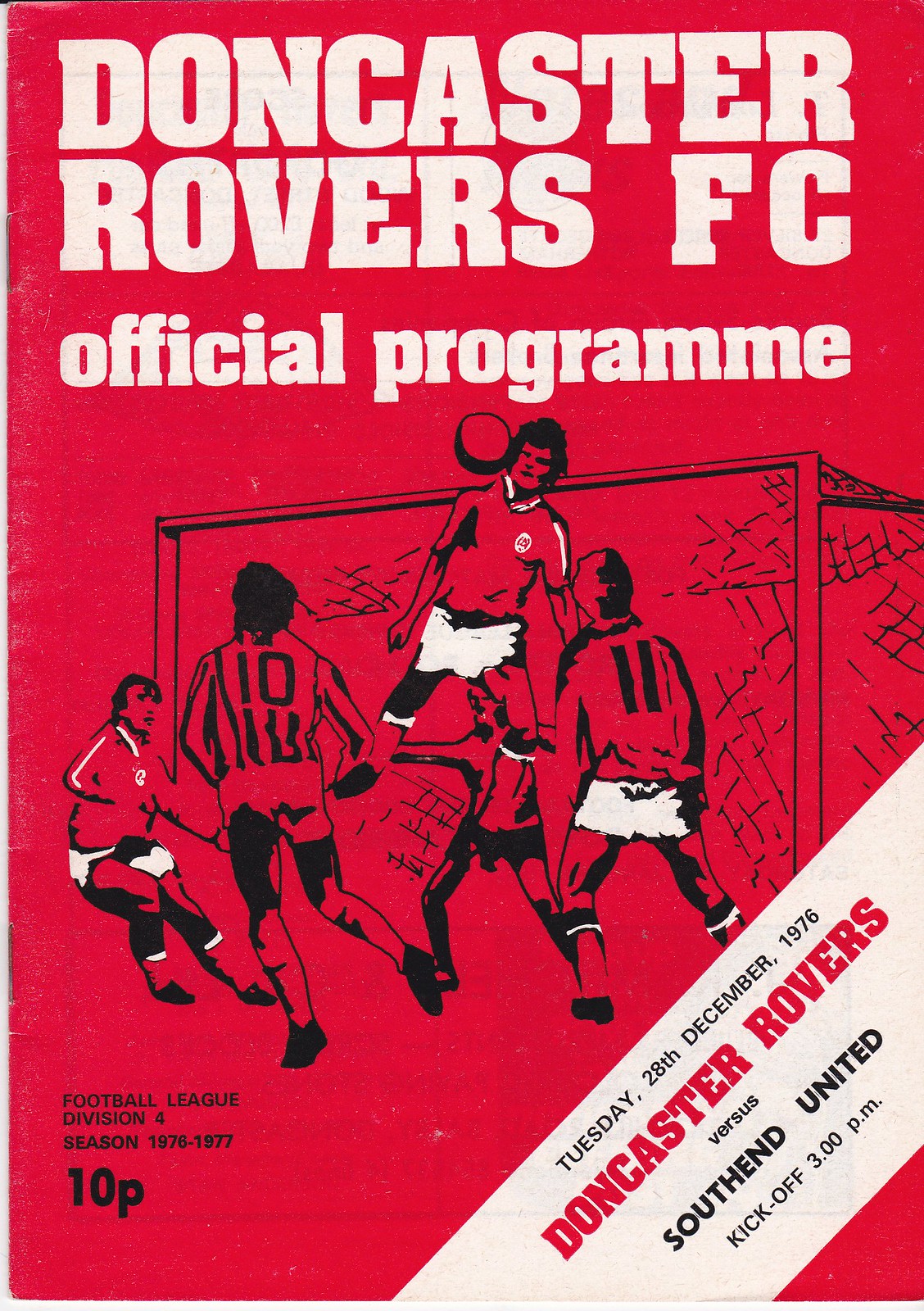The cover of the Doncaster Rovers FC official program from the 1976-1977 season is designed in a striking red, with the title and other details in white and black. It prominently features a cartoon drawing of players in an intense moment of a soccer game, with a goalie appearing to block a ball near the goal. The program, dated Tuesday, December 28, 1976, announces a match between Doncaster Rovers and Southend United, with a kickoff scheduled for 3 p.m. The vintage 1970s aesthetic is highlighted by the bold use of colors and dynamic illustration, encapsulating the excitement and anticipation of the upcoming game.